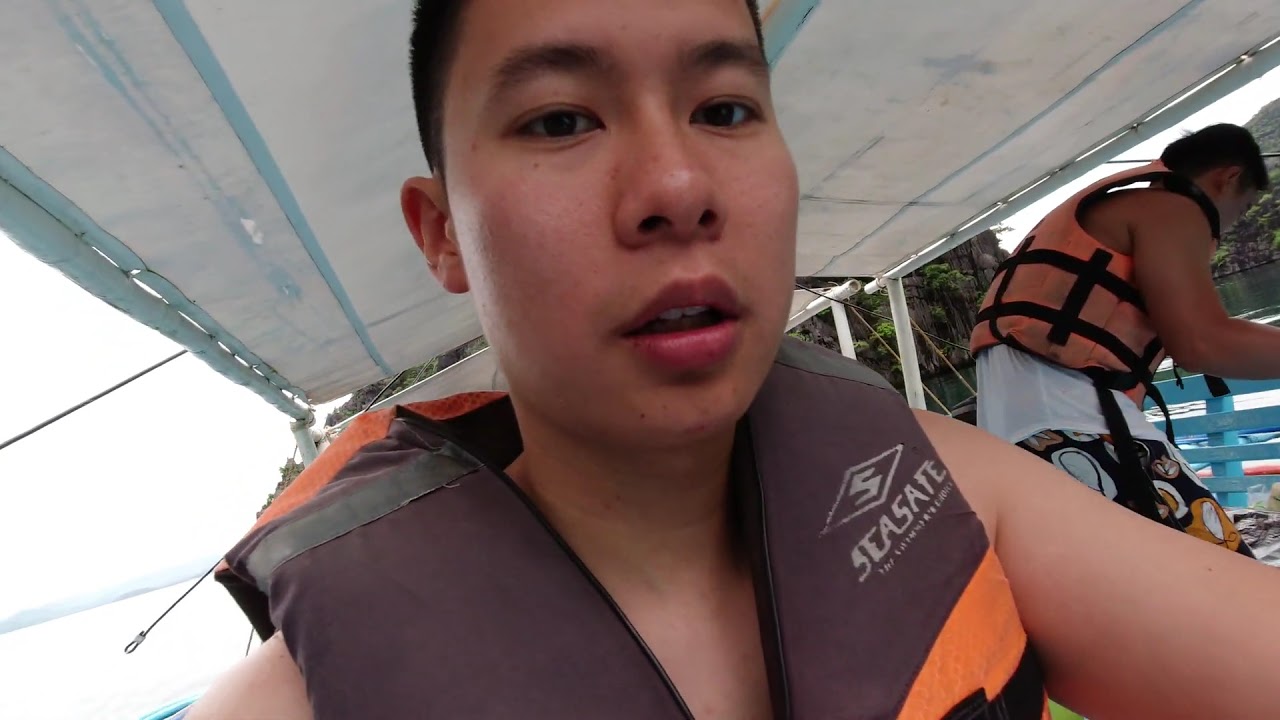The image is a close-up photograph that seems to have been taken on a boat or near the shore. At the center of the photo is a young man, likely a teenager, with short-cropped black hair. He has a tanned complexion and is wearing a dark gray and orange life jacket with a logo that says "Seasafe," accompanied by a diamond shape and an "S" on it. His facial expression is serious, looking down at the camera, possibly indicating that this may be a selfie. 

To the right of the main subject, in the background, is another young man with dark hair. He is seen from the back and is wearing an orange life jacket over a white tank top and patterned black shorts. He appears to be bending over, pretending to do something. 

Above them, there's a white canopy with blue trim, hinting that they are on a vessel. The background is overexposed and somewhat blurred, but you can make out rocks and an overcast sky, adding context that they might be near water or on a boat by the shore. The left corner of the image also shows a glimpse of water, further suggesting the proximity to a waterfront.